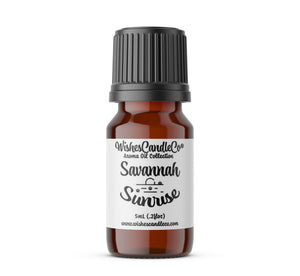The image features a small amber glass bottle with a shiny finish and a black cap. The bottle is labeled with a white tag that reads, "Wishes Candle Co." at the top, followed by "Savannah Sunrise" in smaller print. The label includes a hand-drawn black illustration of a sun rising over a horizon and states the bottle's volume as five milliliters. Below the volume, the website to purchase the product is printed. The bottle appears to contain an essential oil or an aroma oil from the "Aroma Oil Collection," which gives it a reddish-brown appearance. The image is set against a plain white background with no additional elements or backdrops, making it look like a staged product photo typically used in advertisements.